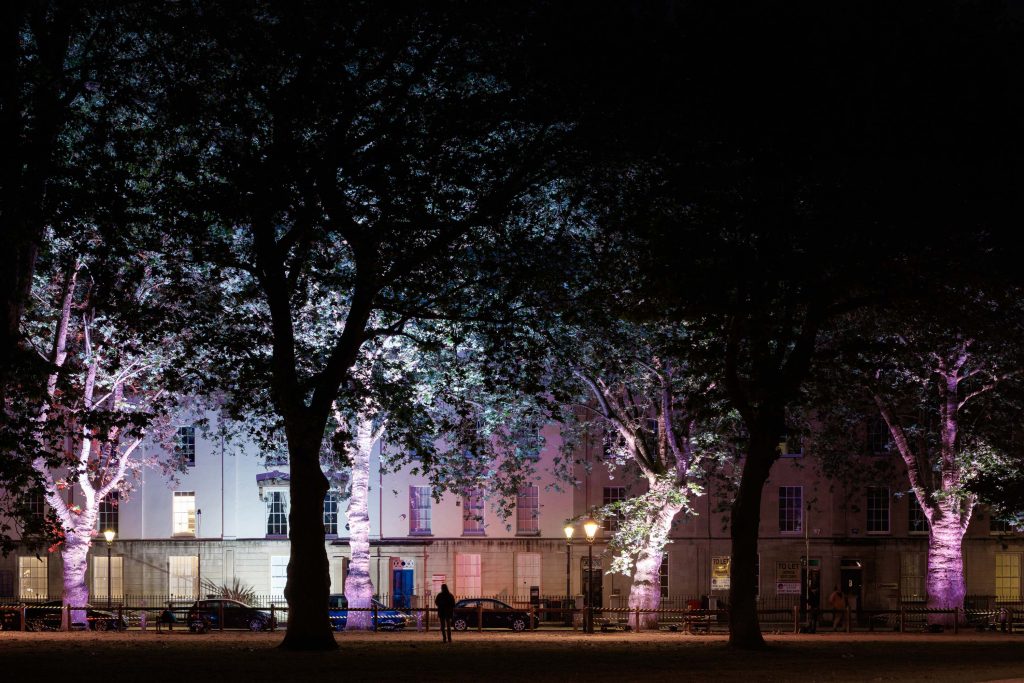This nighttime photograph captures a striking scene dominated by a large white building in the background, partially obscured by tall mature trees with dense foliage. The trees are silhouetted in the foreground, appearing completely black, while several trees in the midground are dramatically lit with purplish-white lights, likely from ground lamps. These illuminated trees cast a subtle glow that accentuates their leaf outlines against the dark sky. The house, grand and imposing, features numerous windows, some of which are lit up, emitting a soft white light. At the very bottom of the image, a person and several cars, dwarfed by the building's size, along with a stone wall or small fence in front of the house, add a sense of scale. The combination of natural and artificial light creates a captivating contrast, enhancing the photograph's overall depth and atmosphere.